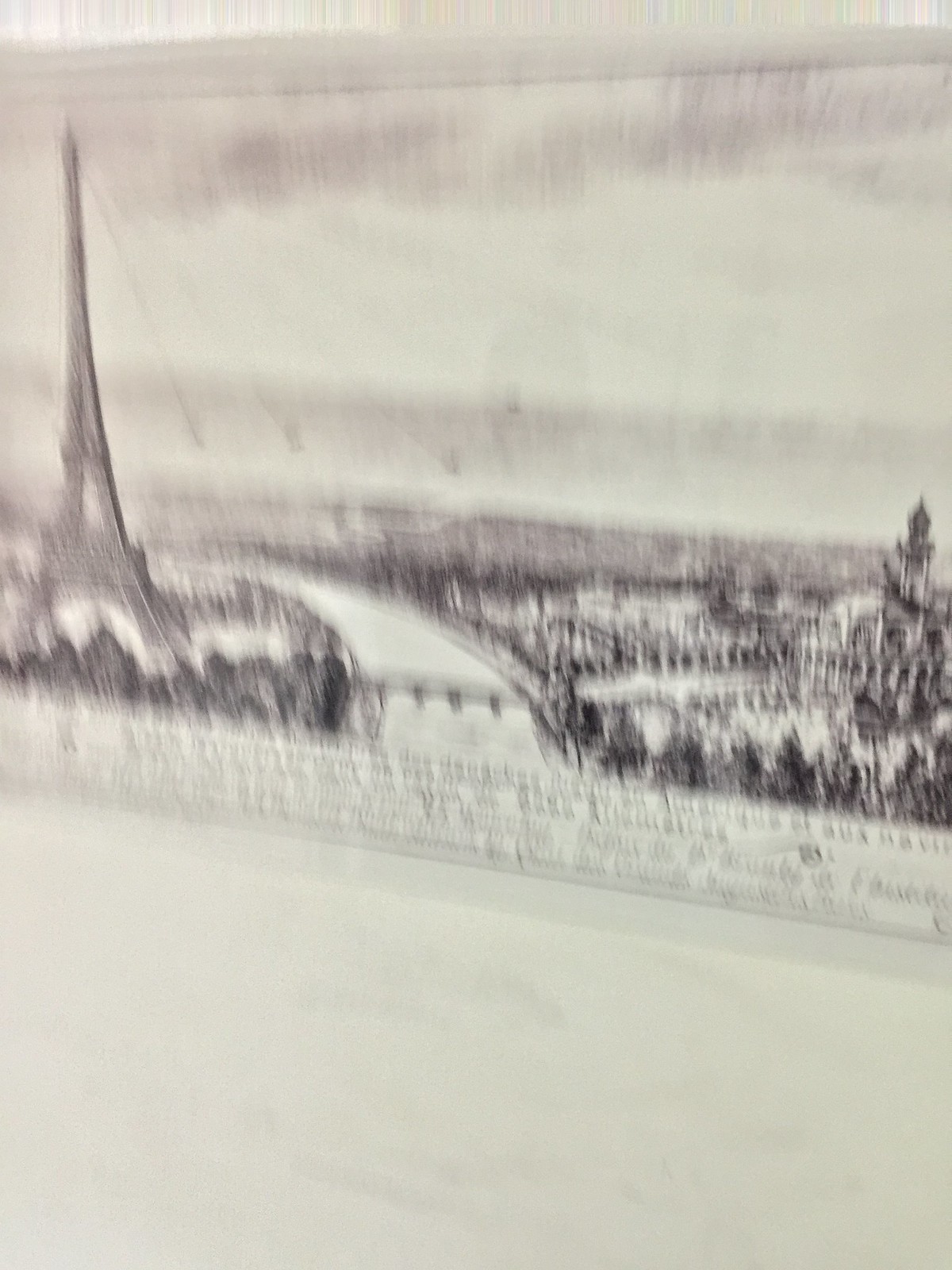A detailed pencil sketch captures a serene daytime scene of the iconic Eiffel Tower. The vantage point appears to be from a bridge over the River Seine, looking eastward. The Eiffel Tower is prominently visible to the left, or north, of the river. The sketch is composed of shades of gray, black, and off-white, emphasizing the intricate details of the tower and its surrounding landscape. The bridge, which crosses the river at the base of the Eiffel Tower, is depicted in a pure white or slight off-white, providing a stark contrast to the rest of the artwork. In the background, the cityscape appears to be from a bygone era, with no modern high-rises cluttering the view, harkening back to a simpler time in Parisian history. The overall composition of the drawing gives a nostalgic glimpse into the past, beautifully capturing the essence of Paris in a monochromatic palette.